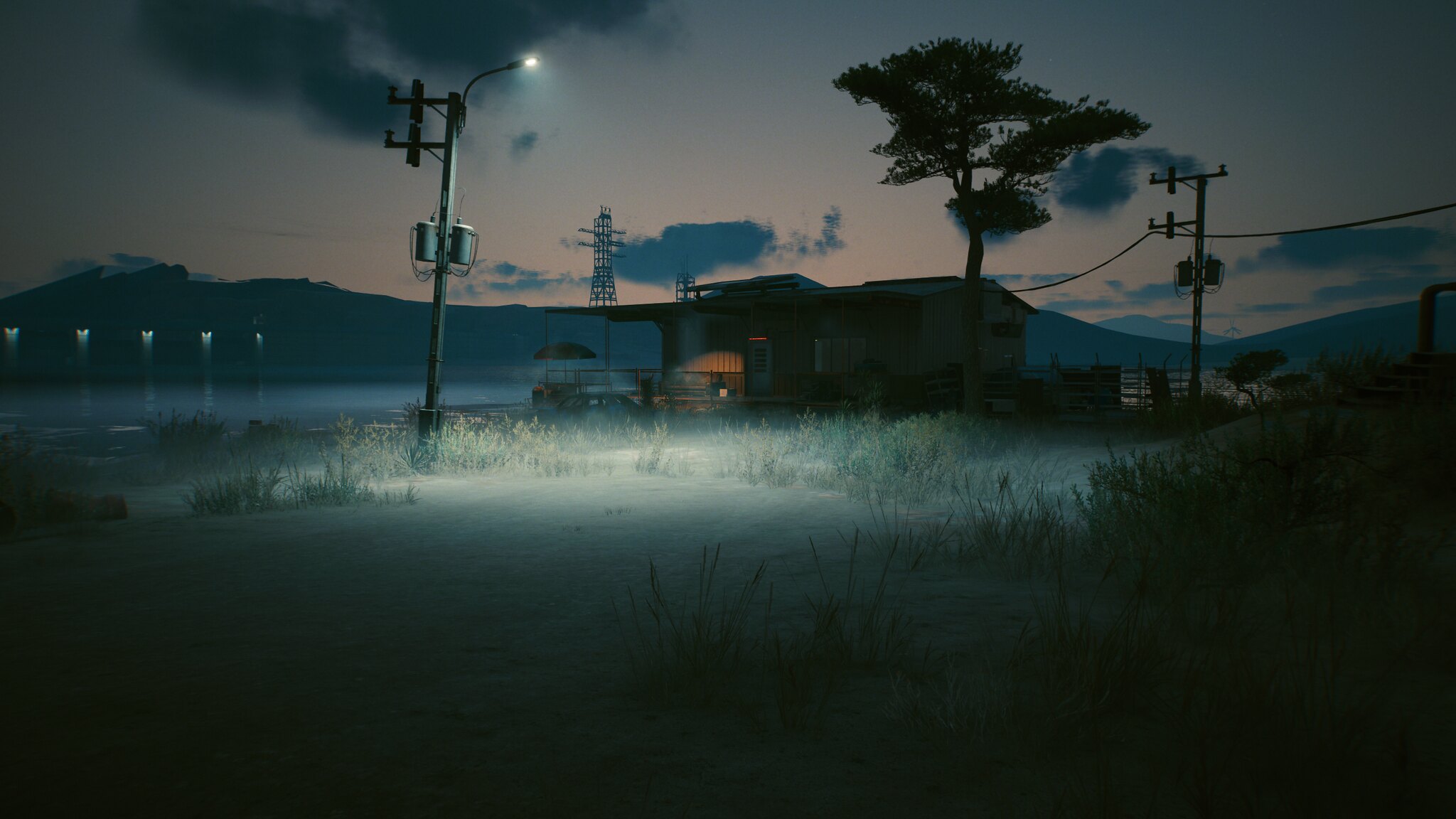In this rural scene, a solitary streetlamp casts a warm glow on a patch of soil, illuminating tufts of long grass scattered throughout. Surrounding the area, a wooden fence delineates what appear to be animal enclosures, adding to the rustic charm. Nearby, a shed-like structure with robust metal sheet roofing stands, suggesting a barn or storage building, adding a touch of agricultural functionality. In the backdrop, a majestic mountain range stretches across the horizon, while a tall tree stands sentinel next to the metal-roofed shed, its branches reaching skyward. Adding to the infrastructure are power lines stretched taut between imposing poles, and a towering metal power tower further enhances the scene, hinting at human presence amid the natural and pastoral elements.